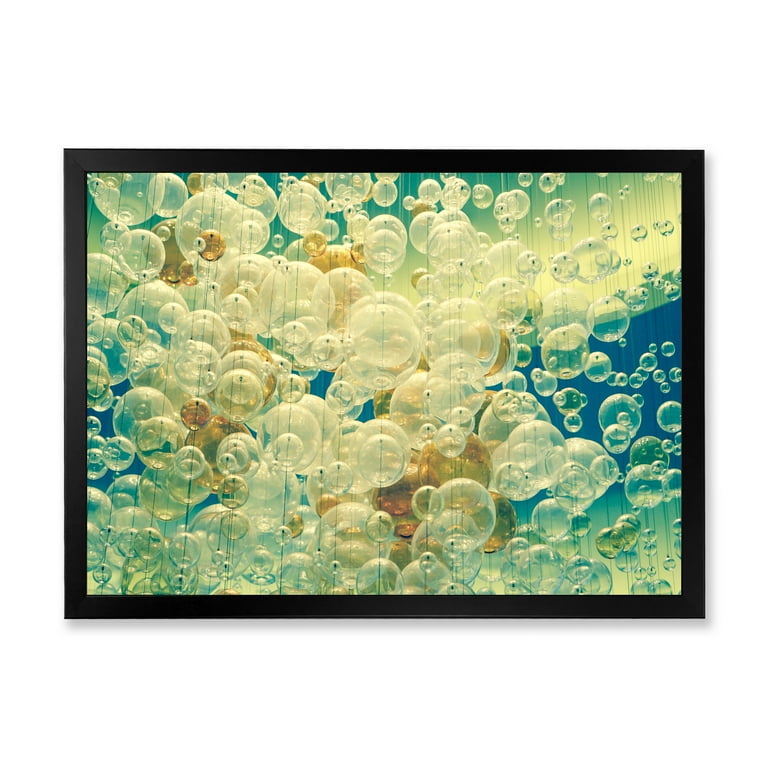The framed painting features a highly imaginative, surreal depiction of bubbles, accentuated with a 3D effect, possibly created using acrylic paints. Housed within a simple, thin black frame, the scene presents an array of bubbles varying from clear to nearly clear, extending to greenish and amber hues. These bubbles, of all different sizes—ranging from large to tiny—appear to be suspended in mid-air, seemingly attached to vertical strings or wires. The predominant colors in the painting include a rich medium ocean blue background with contrasting white, green, and amber highlights. Particularly, some bubbles exhibit dots, and gold or tan bubbles are clustered towards the upper left portion. The painting is bathed in natural light, which enhances the surreal and imaginative essence of the scene.